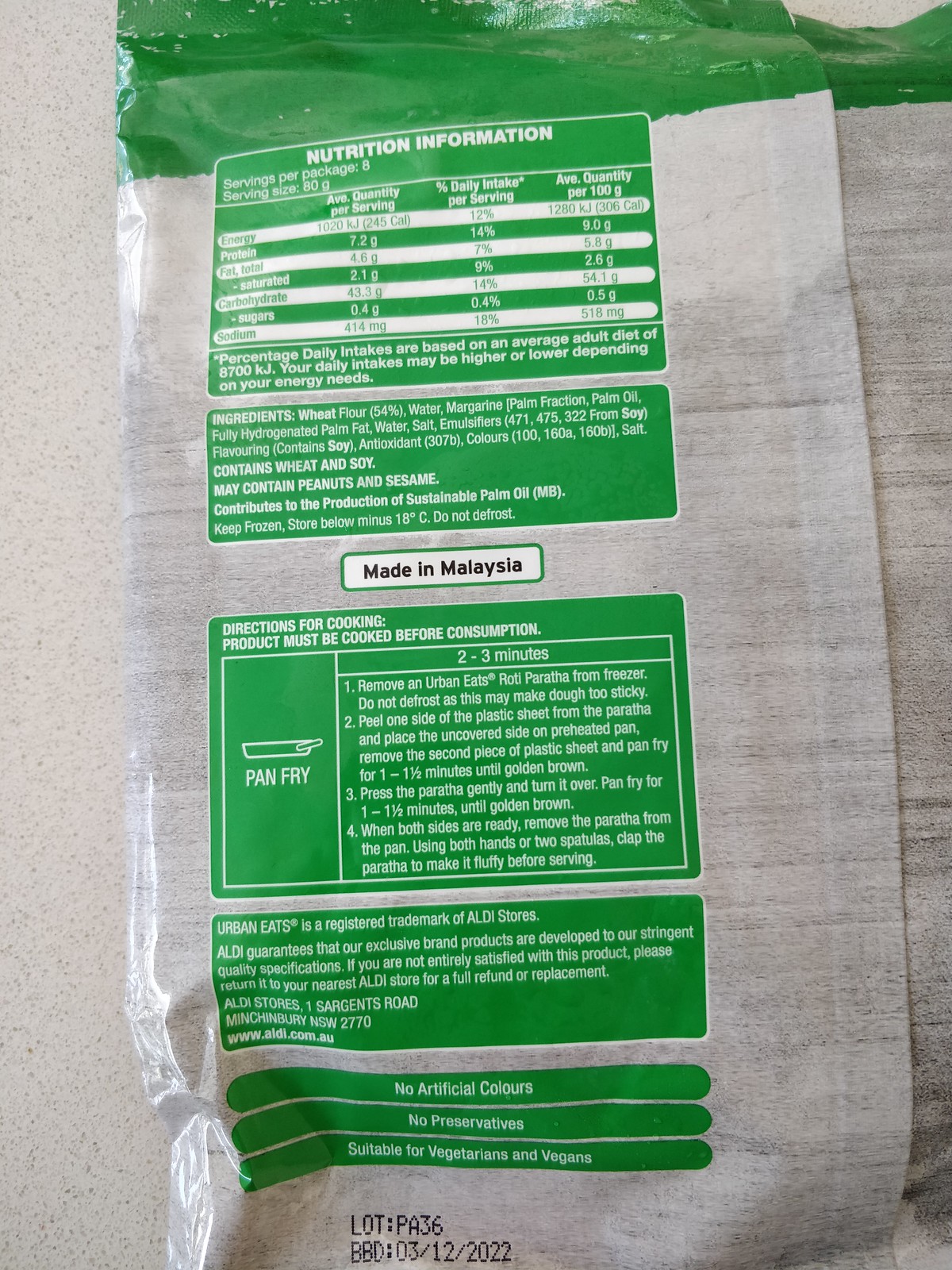The image features a gray background showcasing two packages. Each package is primarily gray, adorned with various green boxes. One of the green boxes is labeled "Nutritional Information" in gray writing, detailing the nutritional content of the product. Adjacent to this is another green box with light gray text listing the ingredients. Additionally, a small green box with a white interior prominently states "Made in Malaysia" in black letters. Further down, additional green blocks provide cooking instructions, including steps for pan-frying the product.